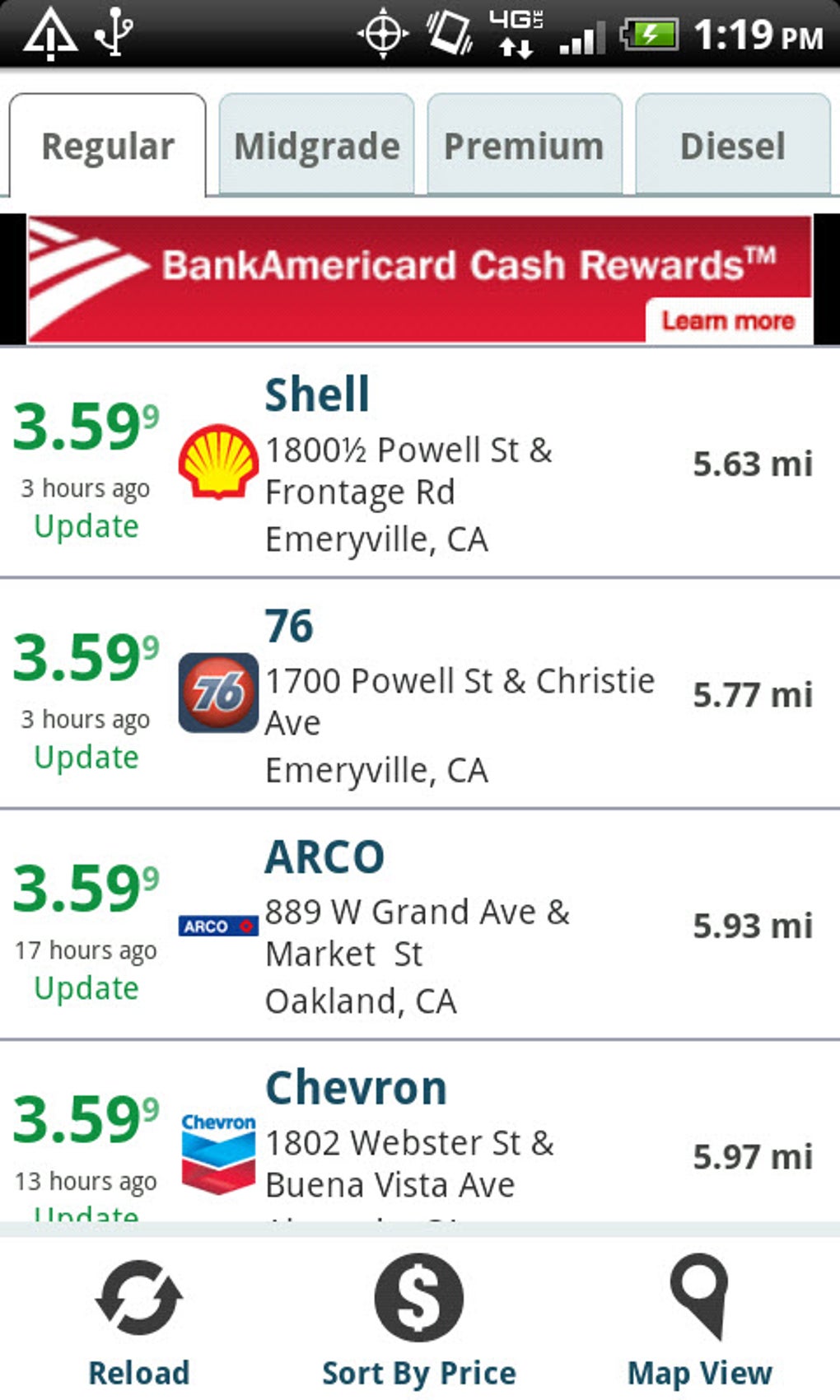This image, captured from a cell phone screen, displays a detailed list of gas prices at various stations. At the top of the screen, options for fuel types are visible, including Regular, Mid-Grade, Premium, and Diesel. A prominent red banner at the top promotes the Bank AmeriCard Cash Rewards program with a clickable "Learn More" section.

The prices begin with a Shell station in Emeryville, California, showing Regular gas at $3.59 and 9/10ths of a cent, updated three hours ago. The same price of $3.59 and 9/10ths of a cent is listed again for a '76' gas station, also in Emeryville, California, with the same update time of three hours ago.

In the next row, an Arco station in Oakland, California, is listed with the identical price of $3.59 and 9/10ths of a cent. Finally, a Chevron station located at the intersection of Webster Street and Buena Vista Avenue, 5.97 miles from the current location, lists its prices at $3.59 and 9/10ths of a cent, updated 13 hours ago.